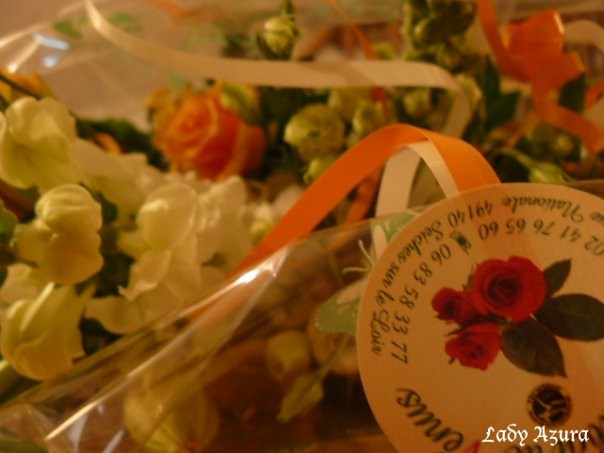This image is a color photograph of a close-up bouquet of flowers, wrapped in clear cellophane, which makes the details slightly obscured and out of focus. Dominating the upper left-hand corner are white petals, below which lie some peach petals, possibly from a rose. Green foliage can be seen, though specific details are challenging to discern. An orange and white ribbon is curled and laid across the upper right-hand corner and towards the middle of the image.

In the upper right, a round, white sticker featuring red roses surrounded by three leaves is present. The sticker contains numbers, including "024176650," "0683583377," "49140," and text that seems to be non-English, possibly French, making it difficult to read. Additionally, there is an illustration of a cell phone on the sticker.

Wrapping down and around the bouquet is a ribbon or possibly thread, emerging from some packaging located at the bottom right corner of the image. The colors in the photograph include black, white, red, green, orange, pink, light green, tan, and off-white. Notably, superimposed at the bottom right of the image is white text in an old-looking Gothic font that reads "Lady Azura." The setting appears to be indoors, likely during a celebration.